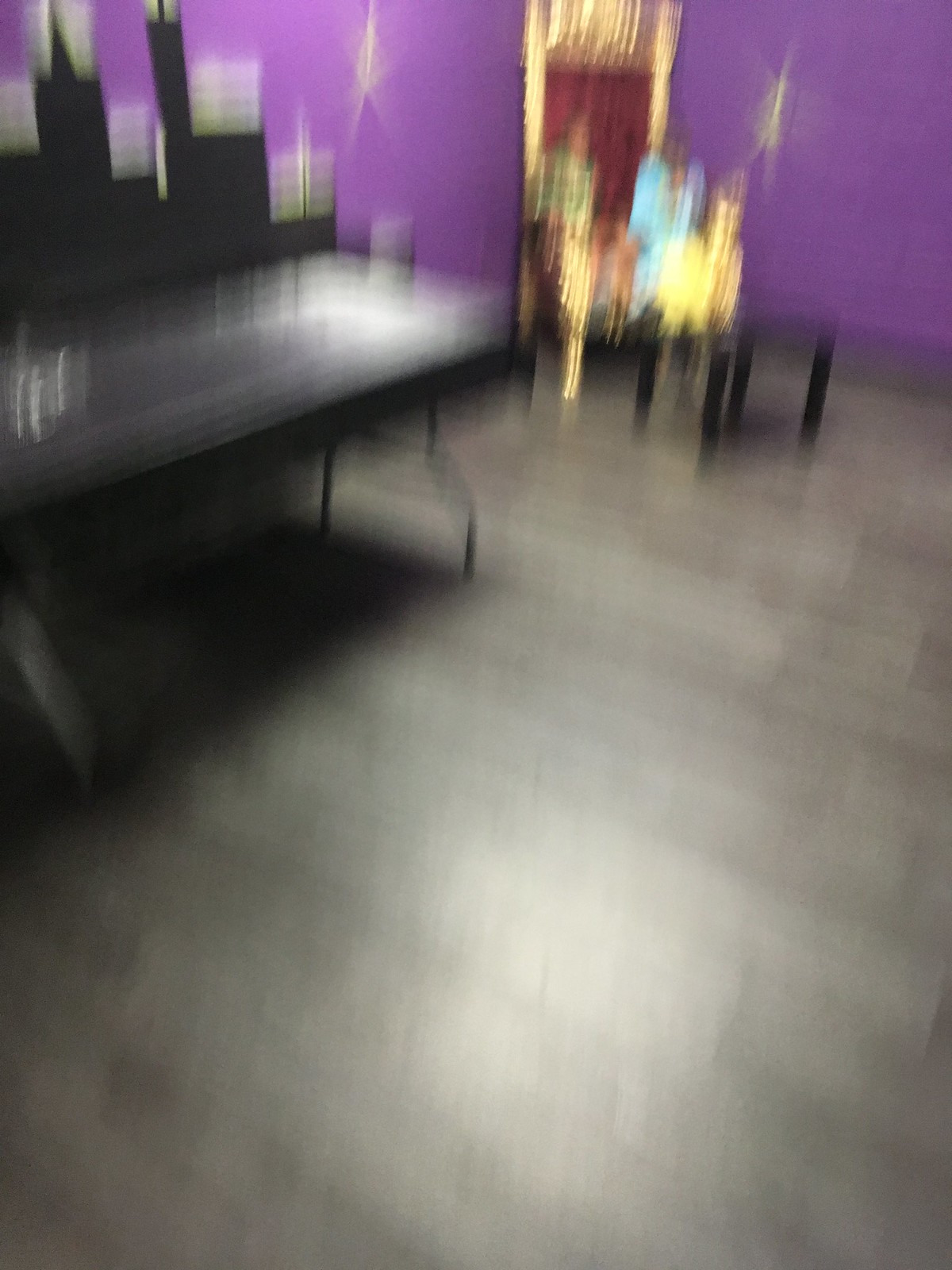The image is an extremely blurry, vertical rectangular photograph of an interior space that appears to be a dance hall. Dominated by bright purple walls in the background, the scene features a large open space with a light tan-gray wooden floor. In the top right corner, an illuminated maroon or burgundy section can be seen, potentially the corner of a room with a chair or a set of statues placed in front of it. The edges of this area are highlighted, and there are shapes that might be people or statues dressed in light blue and green.

A long, black table with metallic legs, running from the center left edge towards the back of the room, lends structure to the otherwise abstract scene. There appears to be something on the table, flanked by shadows below it. 

At the back of the room, a golden-framed doorway set in the purple wall frames a possible entrance. The doorway is accompanied by multiple shapes, potentially depicting two adults and several children entering. One of the adults seems to be wearing turquoise. The wall surrounding the entrance may also feature golden accents and star-like decorations, as well as tall black rectangular shapes that mimic a cityscape.

Overall, the scene reveals a mix of brown, black, purple, gold, and maroon colors, creating a complex, albeit out-of-focus, depiction of what might be a dance hall's interior.